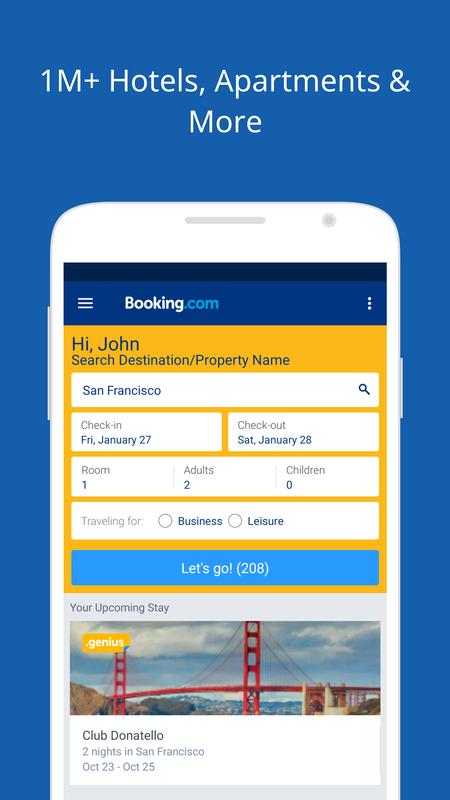**Detailed Caption:**

This image features a vertical layout reminiscent of a typical smartphone interface but without any Android or iPhone symbols. The background is blue, setting a clean and professional tone. At the very top, the text "1M+ Hotels, Apartments, and More" is displayed prominently. Below this heading, there is a detailed computer-generated image of an iPhone displaying the Booking.com app against a white frame.

Inside the depiction of the iPhone, the top bar is blue and displays the Booking.com logo. Beneath the logo, there is a gold rectangular area with the personalized greeting "Hi John" in black text. The text "Search destination/property name" appears below in the white search bar, which shows a typing cursor with "San Francisco" being entered. A magnifying glass icon is situated to the right of the search entry.

Further down the interface, you see input boxes for "Check-in" with the date "Fri, January 27" and "Check-out" with the date "January 28," both in blue text. Below these dates, there are three columns within a long white box, each separated by thin gray lines. These columns are labeled "Room - 1," "Adults - 2," and "Children - 0" in gray text.

Continuing downward, there is another long white box allowing users to select whether they are traveling for "Business" or "Leisure" by checking corresponding circles next to each option in gray and blue text. Below this section, a long blue, clickable box with white text reads "Let's Go (208)."

Moving lower in the image, there is a gray area indicating an "Upcoming Stay." A rectangular photo of the Golden Gate Bridge under an overcast sky occupies this section. In the top left corner of the photo, a gold oval with the word "Genius" in white text is visible.

Below the picture of the Golden Gate Bridge, there is a white rectangle with black text indicating "Club Donatello," followed by the details "Two nights in San Francisco, Oct 23 - Oct 25" in gray text. Judging by the layout and elements, this appears to be a promotional display for Booking.com, inviting users to book their upcoming trips.